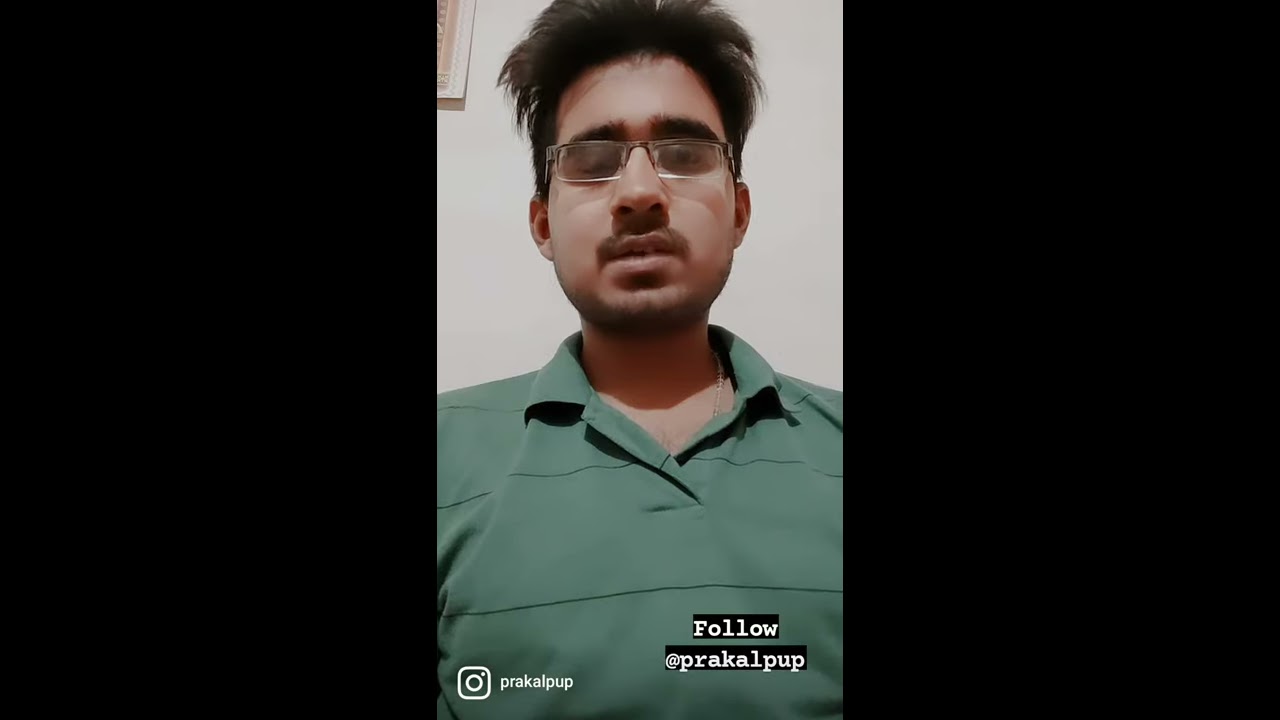The photograph features a young Indian man with clear glasses and distinctive spiky hair, which is short on the sides and tall on top. He has dark brown hair, bushy eyebrows, a thin mustache, and some facial hair on his chin. The man is looking down slightly at a camera that appears to be positioned around his midsection, presenting a focused and somewhat neutral expression with his mouth slightly open. He is engaged in what appears to be an Instagram livestream, as indicated by the white text on the screen, which reads "Follow @Praca1pup" at the bottom, with "Praca1pup" mentioned again to the left. He is dressed in a green collared shirt adorned with wide green stripes separated by thin blue lines, resembling a polo but without buttons. The background is a plain light cream brown wall, slightly obscured by what looks like a faintly visible picture in the upper left corner. The overall setting suggests he is interacting with his audience, possibly giving a talk or performing a skit, as he maintains eye contact with the camera, aiming to engage and potentially grow his viewership.